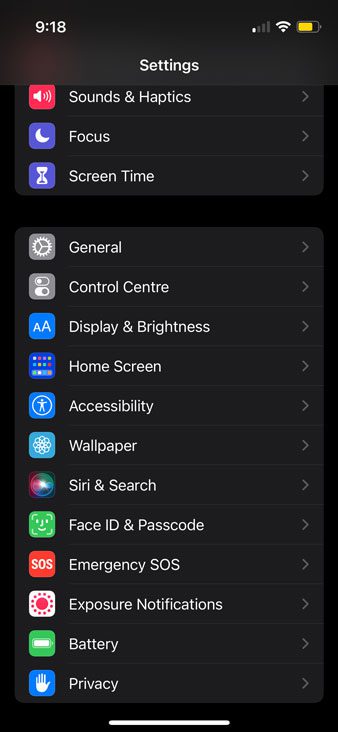The image is a screenshot of a cell phone displaying a settings menu against a black background. At the top left corner, the time is displayed in white text, while the top right corner shows icons for reception, Wi-Fi, and battery status. Just below these icons, centered in white text, is the word "Settings."

The screen is segmented into several horizontal black rectangles, each separated by a light gray line. Each rectangle contains an icon on the left, the name of the setting in the center, and a gray right-pointing arrow on the far right. The first set of options listed are:
- Sound & Haptics
- Focus
- Screen Time

Following a small black gap, the next set of settings include:
- General
- Control Center
- Display & Brightness
- Home Screen
- Accessibility
- Wallpaper
- Siri & Search
- Face ID & Passcode
- Emergency SOS
- Exposure Notifications
- Battery
- Privacy

At the bottom of the screenshot, a thick bright white line is centered horizontally against the black background. This line does not extend to the edges of the screen, maintaining a balanced margin on both the right and left sides.